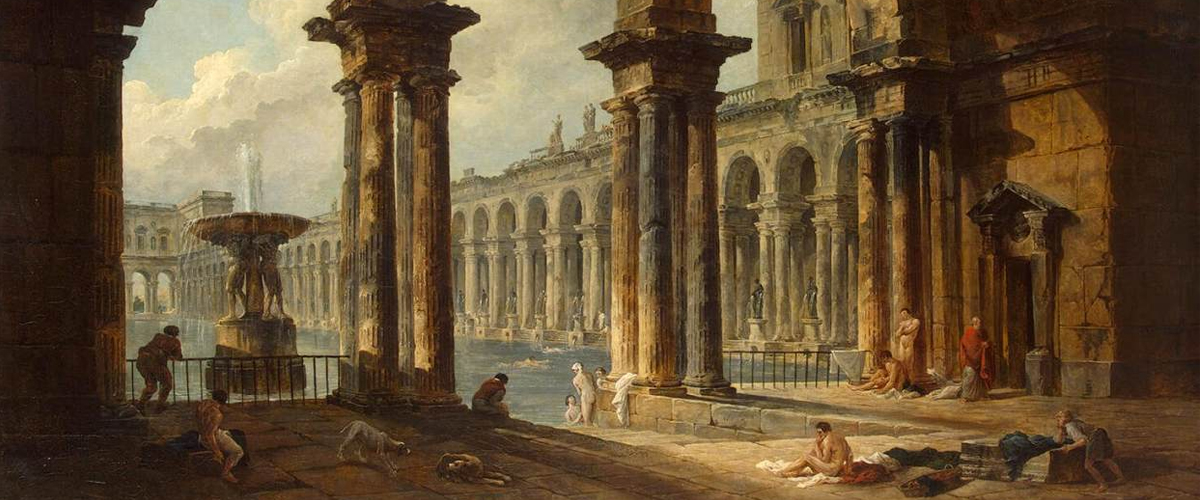This detailed painting by Hubert Robert, titled "Ancient Ruins as Public Baths," depicts a classical scene resembling ancient Roman public baths. Dominating the composition are large classical columns arranged in groups of three or four, creating a long colonnade that extends along one side of the building. The architectural ruins, featuring many arches, stretch from the foreground to the left side of the painting, allowing glimpses of the sky with wispy white clouds in the upper left corner.

In the center of the image lies a large pool of bluish water, accessible by a ramp leading into it. This pool is surrounded by both nude and robed figures. In the foreground, several individuals are depicted lounging on a platform, while others are scattered around the bath, with at least six nude figures visible. Some individuals are on the outer perimeter, dressed in long robes, indicating a historical setting. Moreover, there is a fenced sandbox-like area and a fountain on the left-hand side, adding to the grandeur and everyday life impression of the ancient bathhouse.

Through meticulous details and a blend of ruins and active scenes, the painting vividly brings to life a day at an ancient Roman public bath.